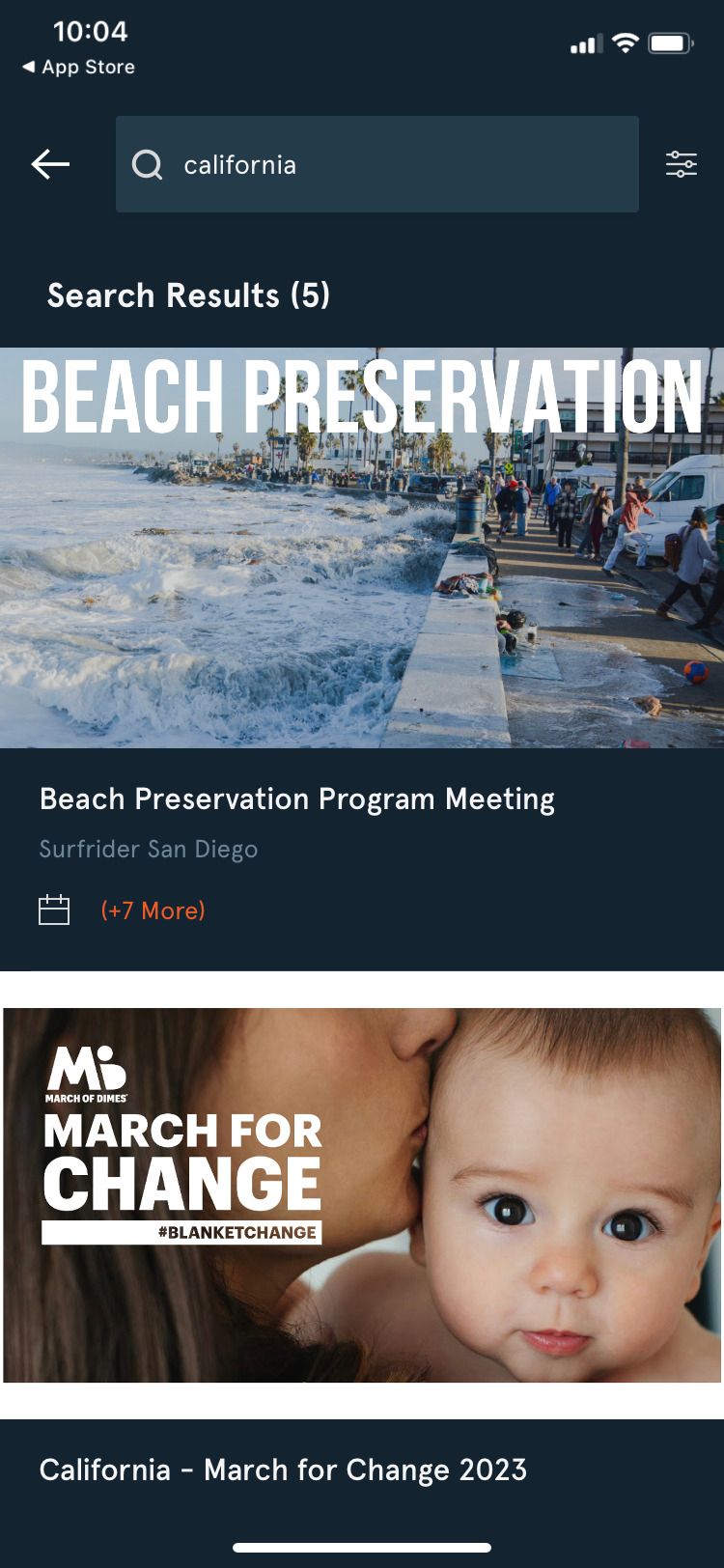**Caption:**

In this image, a search for "California" displays on a smartphone screen, with the filter option visible to the right. Below the search bar, the results indicate five entries. Prominent among these results is an image depicting a dramatic scene at a coastal location. The scene captures a rocky shore with turbulent waters crashing against a concrete retaining wall. People appear to be evacuating the area, frantically running away from the surging waves. A mix of clothing and personal items is strewn about, indicating the urgency of the situation. Several vehicles and blue barrels are also visible in the chaos. 

Further along, the land extends outwards, dotted with additional barrels and palm trees.

Beneath this visual, a textual overlay details a "Beach Preservation Program Meeting" by Surfrider San Diego. An accompanying calendar emoji hints at additional event details (+7 more), marked in orange.

Below this, another event is highlighted with an image of a baby being kissed by a mother, captioned "March for Change" alongside the hashtag #BlanketChange. The logo above this text, an 'M' with a pregnant woman silhouette, signifies the March of Dimes initiative. This section is encased in a dark blue box reading "California March for Change 2023."

At the top of the screen, a standard smartphone status bar shows the time, signal strength for Wi-Fi and phone, battery level, and the option to navigate back or access the app store.